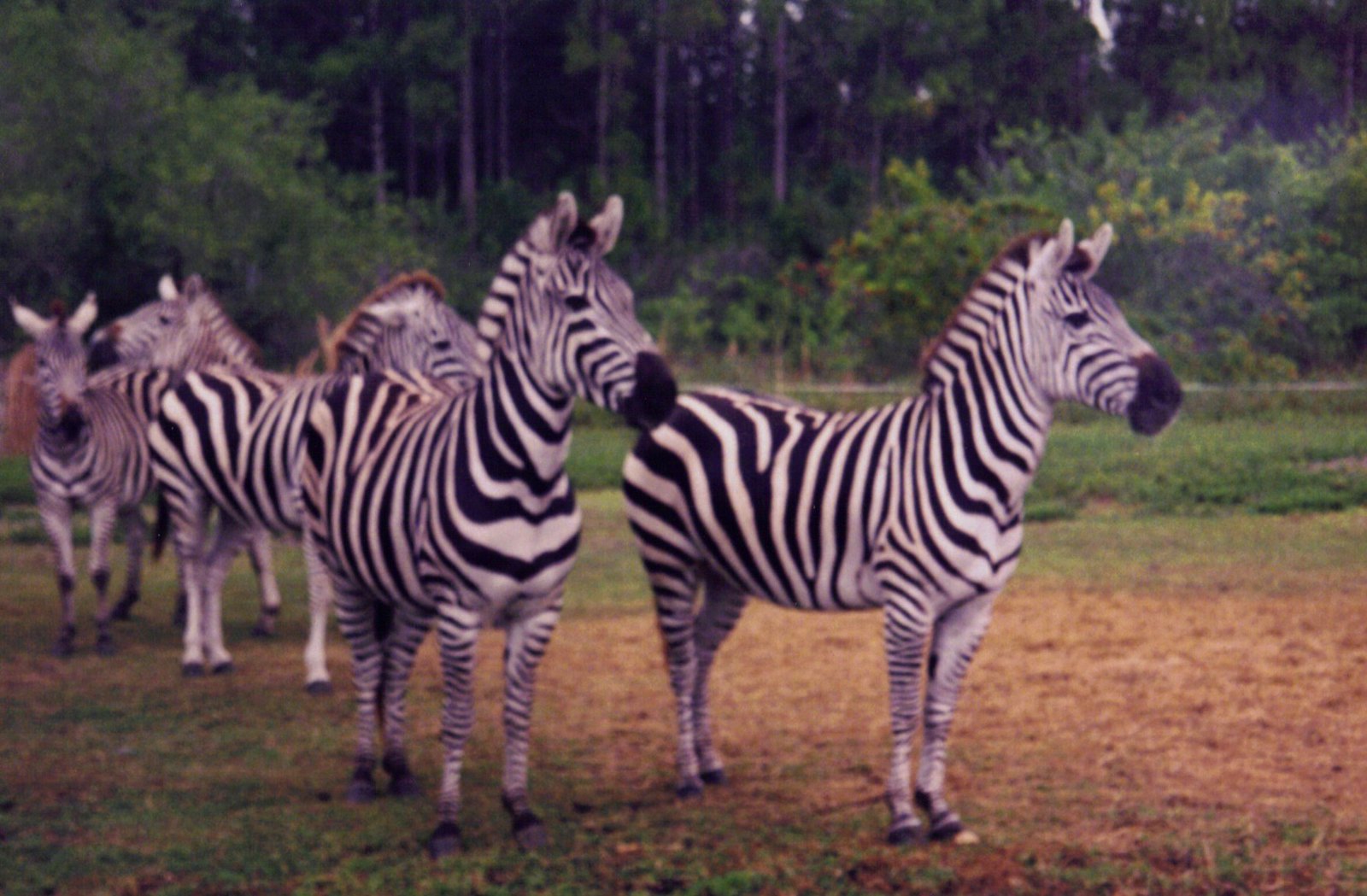The image is a slightly blurred, color landscape photograph depicting a group of zebras standing on a plane of mixed short grass and bare patches. The zebras are arranged in a slightly staggered line, mostly oriented towards the right side of the frame, with one zebra at the back facing left. The scene is set outdoors, heavily suggesting a wild environment, although there is no clear indication of a nature reserve or zoo due to the absence of visible fences. The background features lush greenery with numerous trees and bushes, creating a forested backdrop. The ground towards the front right of the image shows a barren, light brown patch where the grass appears eroded or eaten away, contrasting with the surrounding scattered patches of green grass. There are at least four to six zebras visible, characterized by their striped coats and short manes.